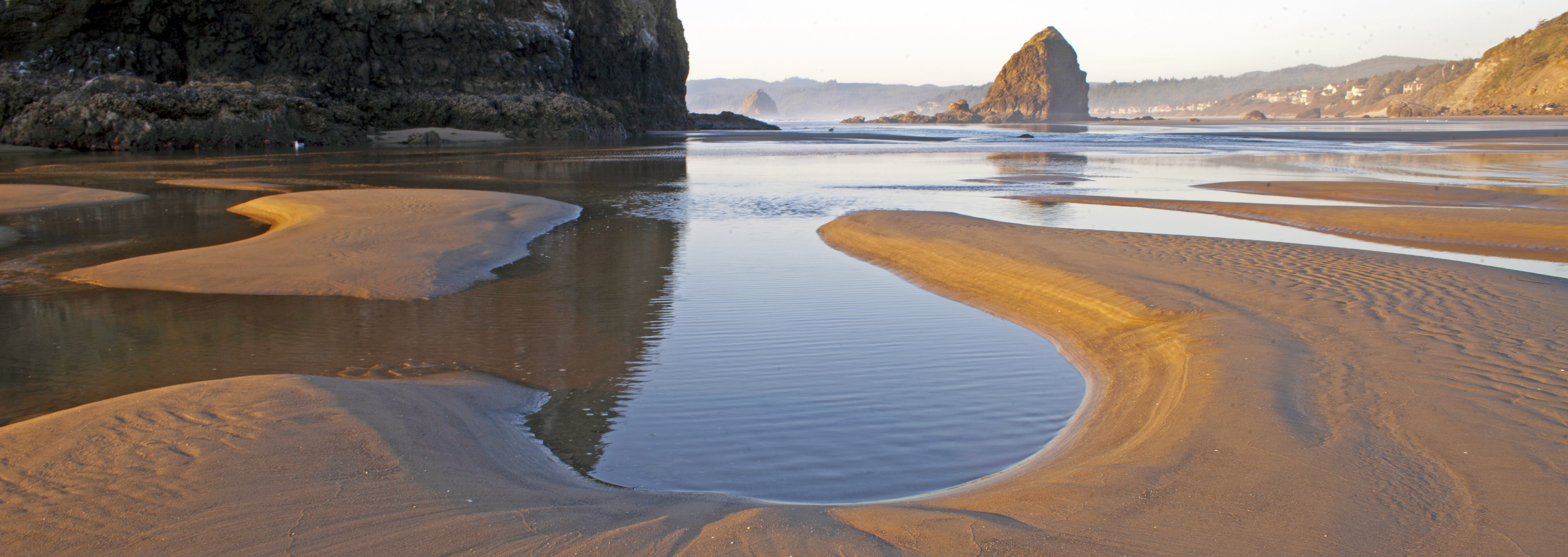The image captures a tranquil coastal scene featuring a series of shallow water bodies and sandbars, forming intricate, sandy shapes and small islands. The water, revealing smooth, flat surfaces interspersed with sandy bottom, remains very calm with mild ripples. The sandy formations curve and intertwine throughout the scene, indicating a secluded cove-like setting. On the far left, a steep, jagged dark gray rock wall rises abruptly, contrasting with the tan-colored sand. Further back, a prominent large rock stands imposingly in the middle of the channel. To the right, a tall, triangular rock structure of the same light sandy color stretches upwards, echoing the surrounding landscape. In the background, another landmass is visible, adding to the enclosed bay-like feel. A gentle yellow cast, likely from the setting sun, bathes the sand and rocks, enhancing the serene ambiance of this coastal tableau.